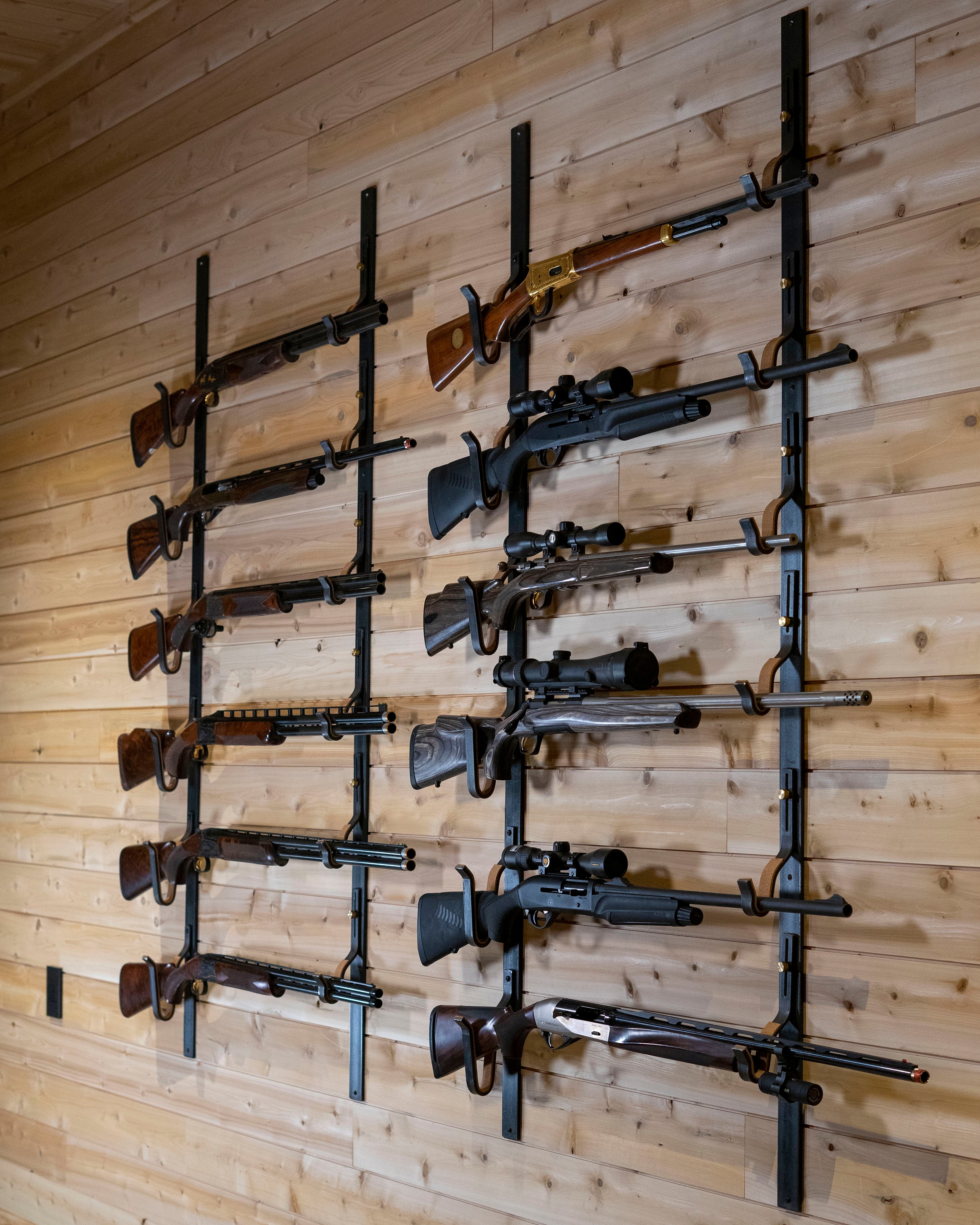This is a vertical rectangular photograph depicting a wall made of horizontally aligned, unfinished wooden planks with visible knots. The wall features two gun racks side by side, both capable of holding six firearms each, constructed from black metal with hooks. The rack on the left holds a uniform collection of shotguns, suggesting they are of a similar type or model. The rack on the right displays a more varied assortment of rifles, including lever-action rifles and those equipped with telescopic sights. The top rifle on the right has a brown stock and appears to be quite old, while the bottom rifle has silver detailing on its sides, indicating its age. Two of the rifles on this rack have scopes, pointing to their potential use for long-distance shooting. In the lower left corner of the image, there is a light switch with a black cover. The floor is not visible in the photograph.